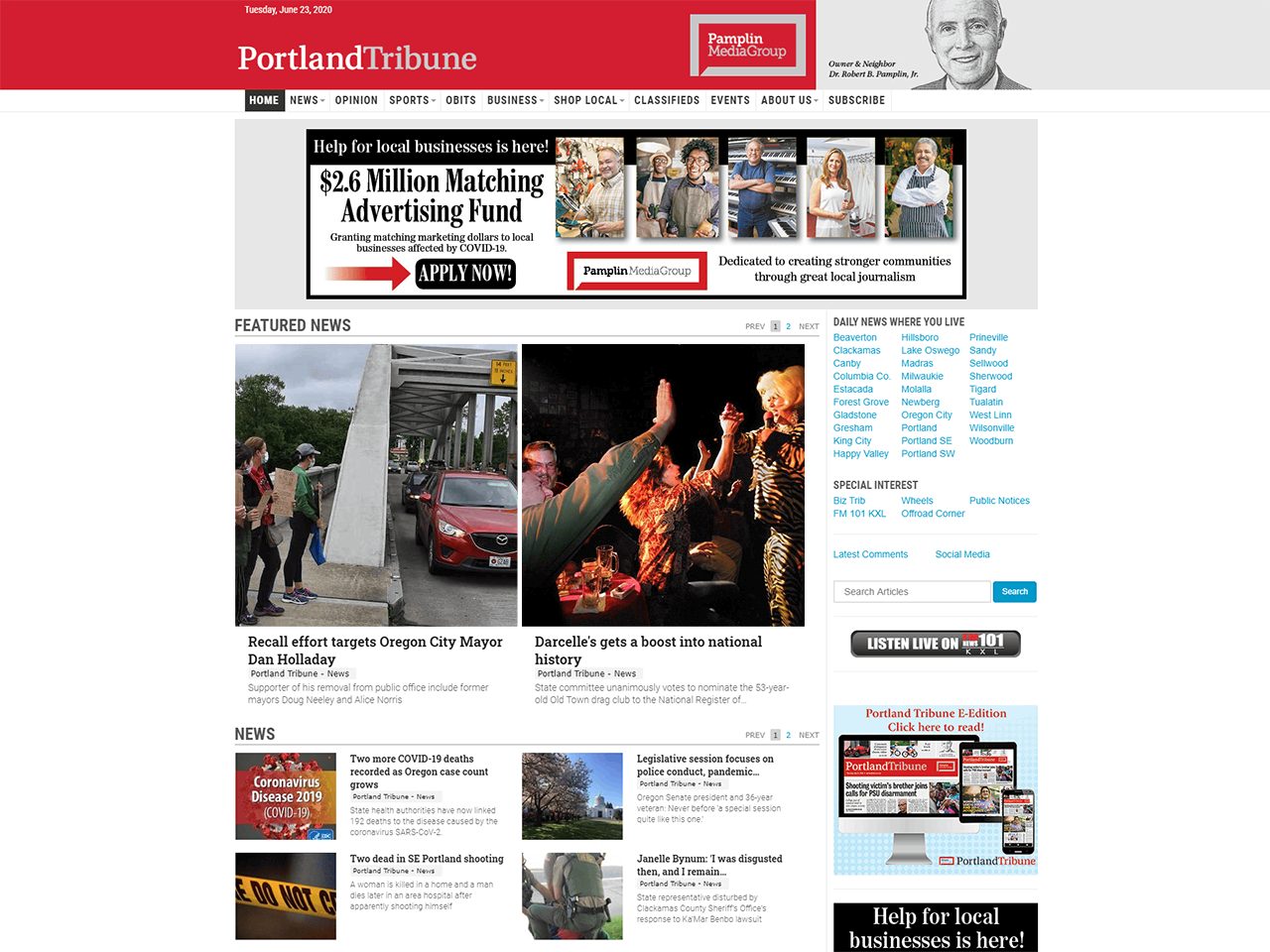The image is a screenshot of the front cover event page of a news website, specifically the Portland Tribune. At the very top, there is a banner that extends from left to right. The left-hand portion of the banner is red and displays the date "Tuesday, June 23, 2020," along with "Portland Tribune" and "Pamplin Media Group" inside a gray box. On the right-hand side of the banner, there is more gray along with an illustration of an elderly man labeled "Owner and Neighbor, Dr. Robert B. Pamplin Jr."

Below the banner is a navigation menu with several items: Home, News, Opinion, Sports, Obits, Business, Shop Local, Classifieds, Events, About Us, and Subscribe. The 'Home' tab is highlighted in white, indicating it is the currently selected page.

Directly beneath the menu, there is an advertisement stating: "Help for Local Businesses is here — $2.6 million matching advertising fund, granting matching marketing dollars to local businesses affected by COVID-19," with a call to action to "Apply Now." 

Further down, there are images of community members accompanied by the text: "Dedicated to Creating Stronger Communities Through Great Local Journalism, Pamplin Media Group."

Finally, a section titled "Future News" features an image of people protesting alongside a bridge with passing cars. The headline reads: "Recall Effort Targets Oregon City Mayor Dan Holliday," followed by "Portland Tribune News."